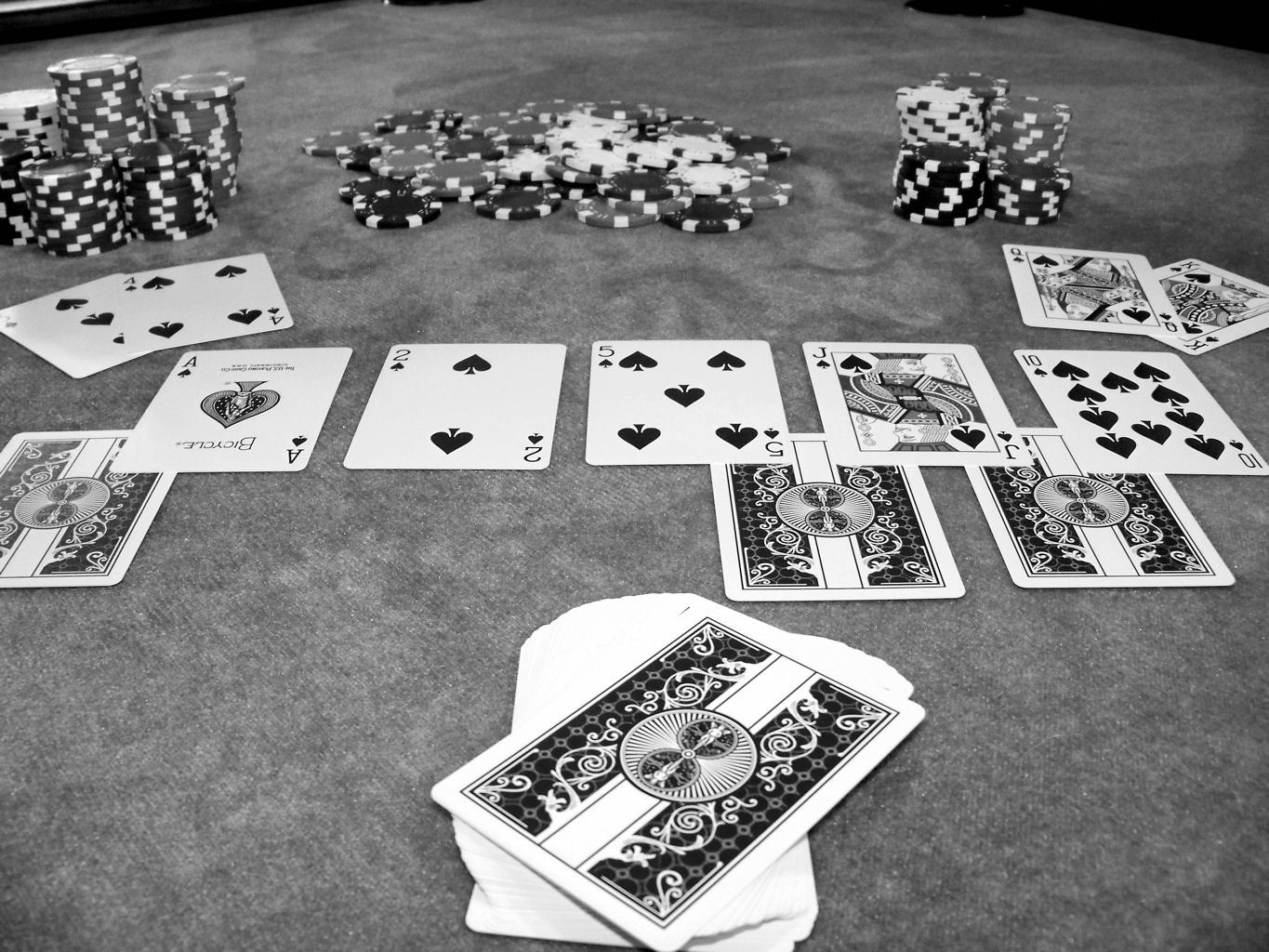This captivating black-and-white photograph captures a high-stakes Texas Hold'em poker game from the point of view of the dealer. At the forefront, a meticulously arranged deck of playing cards forms an elegantly warped pile, curving gracefully to the left and then back to the right, showcasing the edges of each card with precision. 

In the center of the table lies the combination of community cards, revealing a powerful flush: an Ace of Spades, Two of Spades, Five of Spades, Jack of Spades, and Ten of Spades. Adding to the tension, three face-down cards are strategically positioned—two on the right and one on the left—hinting at the hidden potential they hold.

The hands of the players on either side of the table are vividly displayed. The player on the left showcases the Two of Spades and Three of Spades, while the player on the right holds the Queen of Spades and King of Spades, each card adding layers to the strategic narrative unfolding.

Adding a visual rhythm to the scene, stacks of poker chips flank the players' hands on either side, with a formidable pile of chips amassed in the center of the table, symbolizing the intense competition and stakes involved. The photograph beautifully encapsulates the drama and strategy inherent in a poker game, all from the dealer's unique perspective.